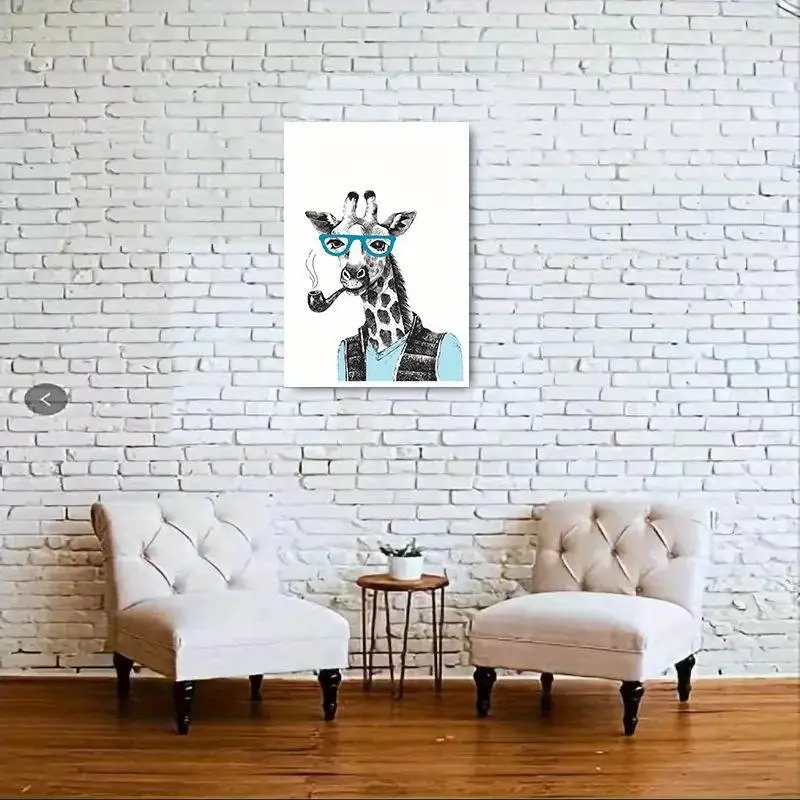The scene depicts a cozy, minimalist sitting area, possibly within an office or business environment. The space features two armless, white cloth chairs with tufted backs designed in a diamond pattern, each with black legs. These chairs are positioned on a medium brown hardwood floor and flank a small brown wooden end table. A green plant, seated in a white pot, adorns the table, adding a touch of greenery. The backdrop is a white-painted brick wall, which may not be genuine brick. Centered on the wall is a vertically oriented, cartoon-style painting of a whimsical giraffe. The giraffe, sporting blue eyeglasses, a seafoam green shirt, and a gray vest, smokes a black pipe with visible smoke trails. This detailed setup combines a charming mix of whimsy and modernity.